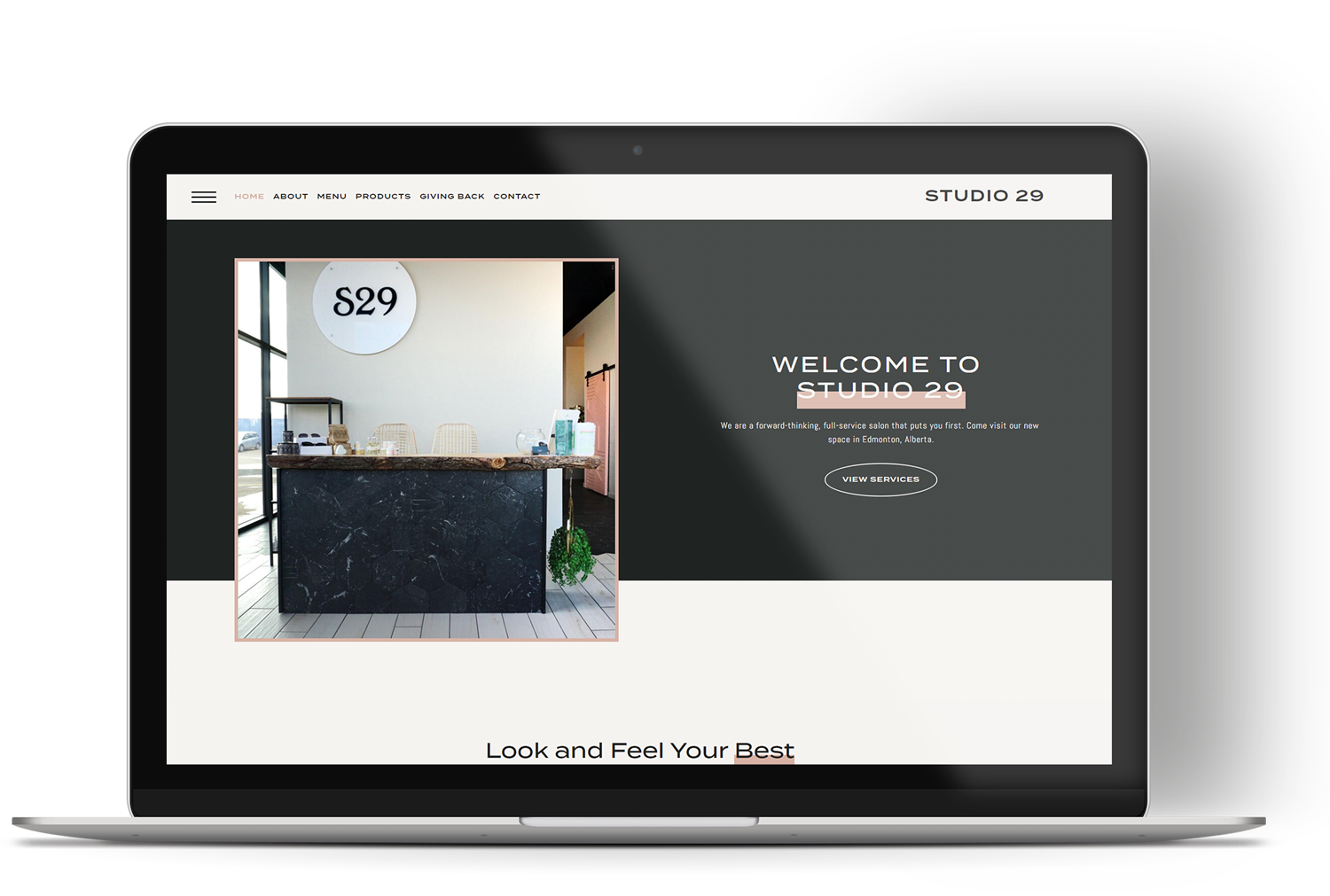The photograph showcases a vertically oriented tablet set on a table, featuring a prominently displayed website on its screen. Framed in black, the tablet has a thick black banner across the top and a white banner at the bottom. The website header, "Studio 29," is visible at the top, with various menu options aligned horizontally along with a hamburger menu on the far left. Just below, a large black banner dominates the screen, containing a welcoming message in white text that reads "Welcome to Studio 29."

On the left side of this banner, there's an insert image resembling a check-in counter or front desk, made of blue granite or marble, likely situated in a professional setting such as an office building. Behind this counter, a white backdrop features a significant circle with the letters "S29" inside, indicative of the salon's branding. 

Further to the right of the insert image, more text is visible under the black banner. Though some smaller pink letters remain unreadable, prominent pink lettering on a banner invites visitors to explore the space, labeling it as "Studio Frontier 29." Below this, an oval within the pink banner contains more text, but it's difficult to discern its content due to its small size.

The bottom portion of the screen is dominated by a white banner displaying the text "Look and feel your best" in gray on a clean white background. The overall depiction of the tablet's screen provides a detailed view of Studio 29's website, emphasizing its welcoming nature and emphasis on customer experience.